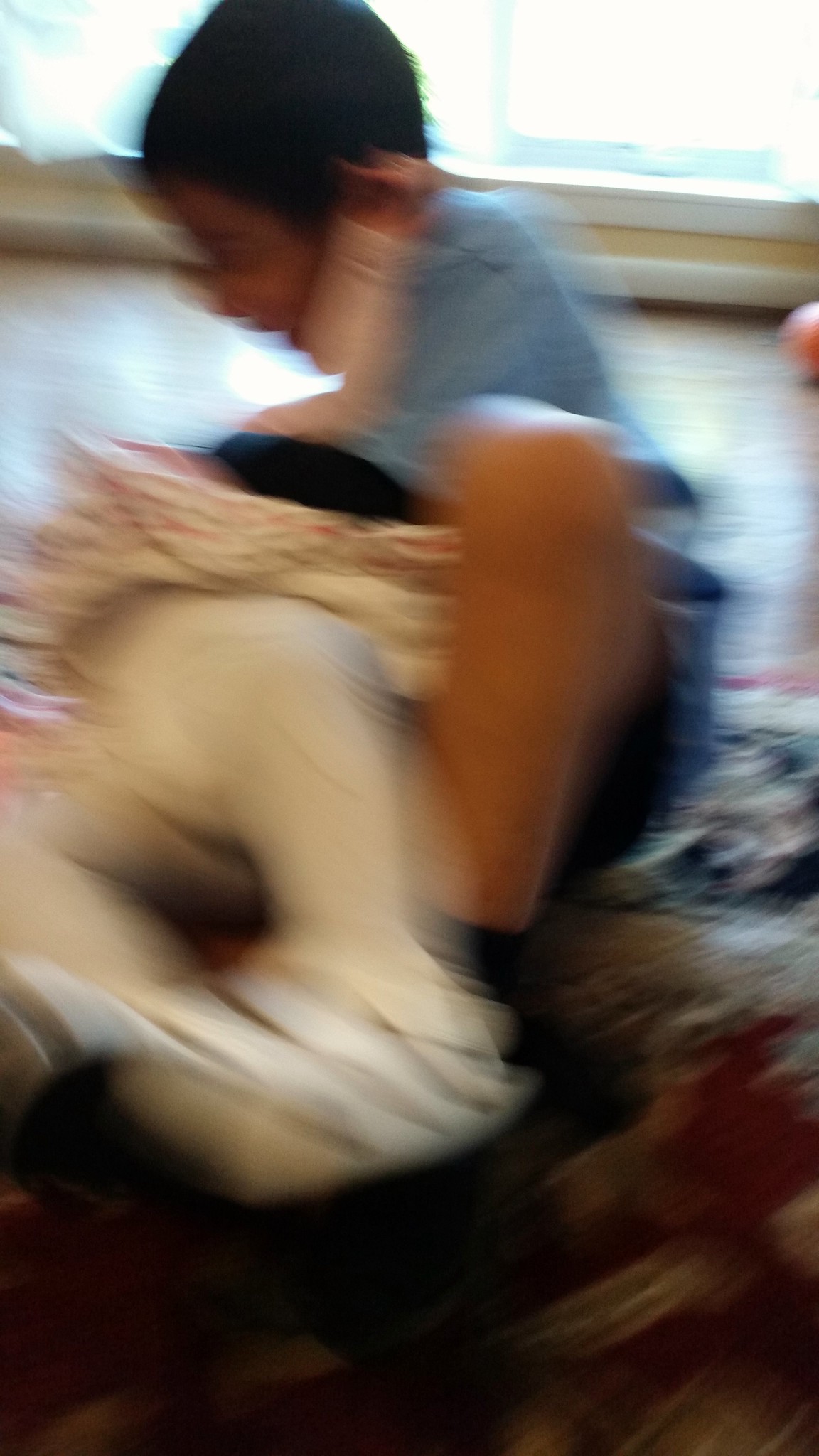In a brightly lit room with yellow and white walls and a wooden floor, two children are captured in a blurry, playful wrestling match. The central focus is on a young boy with black hair and olive skin, dressed in a blue shirt, navy or black shorts, and black socks. He is sitting upright with his left knee raised, his left foot tucked under the other child, and his arms in motion, seemingly engaged in wrestling. The other child, a girl, is perched on his lap, leaned back across his body, and wearing a white and pink floral skirt with white tights. Her face is not visible but her arm is raised near the boy's neck, contributing to the wrestling motion. They are on a patterned area rug with red, black, and possible gold designs. In the right corner, part of another child or person's knee is barely visible. The background features the bright light from a window, a baseboard, and the wooden floor extends out from under the patterned rug.